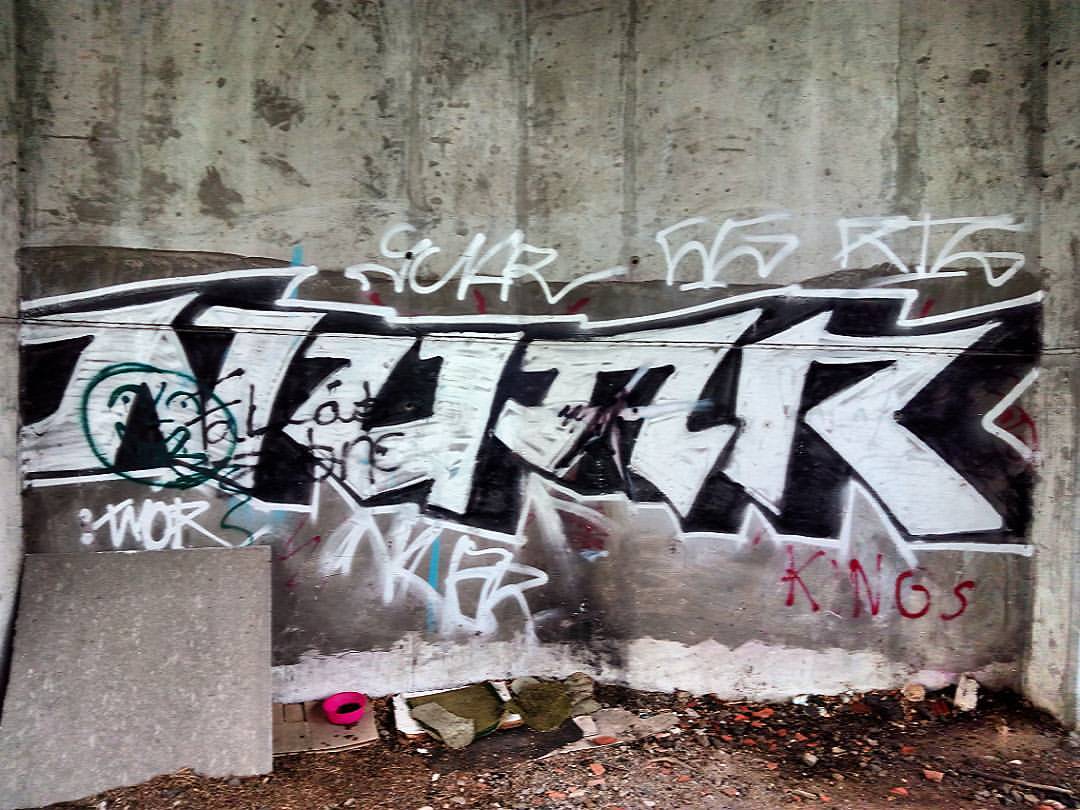This image captures a chaotic graffiti scene on a concrete wall beneath a bridge or overpass. Dominated by large, white letters spelling "N-U-N-R," the graffiti is layered over a black backdrop, which itself is outlined in white. Below these letters, the red spray-painted word "Kings" (possibly "K-N-G-S" due to fading) stands out, albeit sloppily. The graffiti appears to be a mix of tags and scribbles, reflecting a competition for space among various artists. The ground is littered with debris, including a red bowl with something in it, scattered items, and what might be a cardboard piece, suggesting that the area might have been occupied by homeless individuals. The concrete wall also shows patches of greenish discoloration.